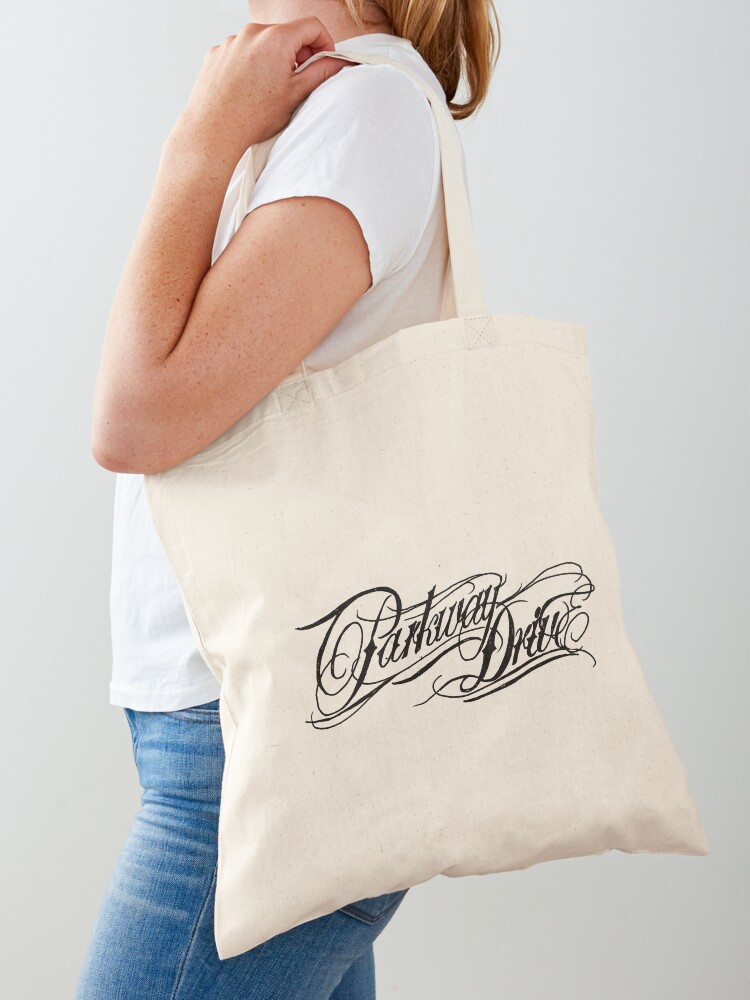This photograph captures a Caucasian woman with shoulder-length, dirty blonde hair, dressed in a short-sleeve white t-shirt and medium-toned blue jeans with some distressing on the thighs. She stands in front of a light gray, almost white, background, and her head is partially cut off, showing only her neck and the lower portion of her hair. Draped over her left shoulder is an ivory-colored canvas tote bag adorned with intricate, fancy black lettering spelling out "Parkway Drive," complete with ornamental whorls, loops, and curvy underlines. The woman holds the tote handle with her left thumb, which is tucked underneath the strap, and the bag appears spacious enough to carry numerous items.